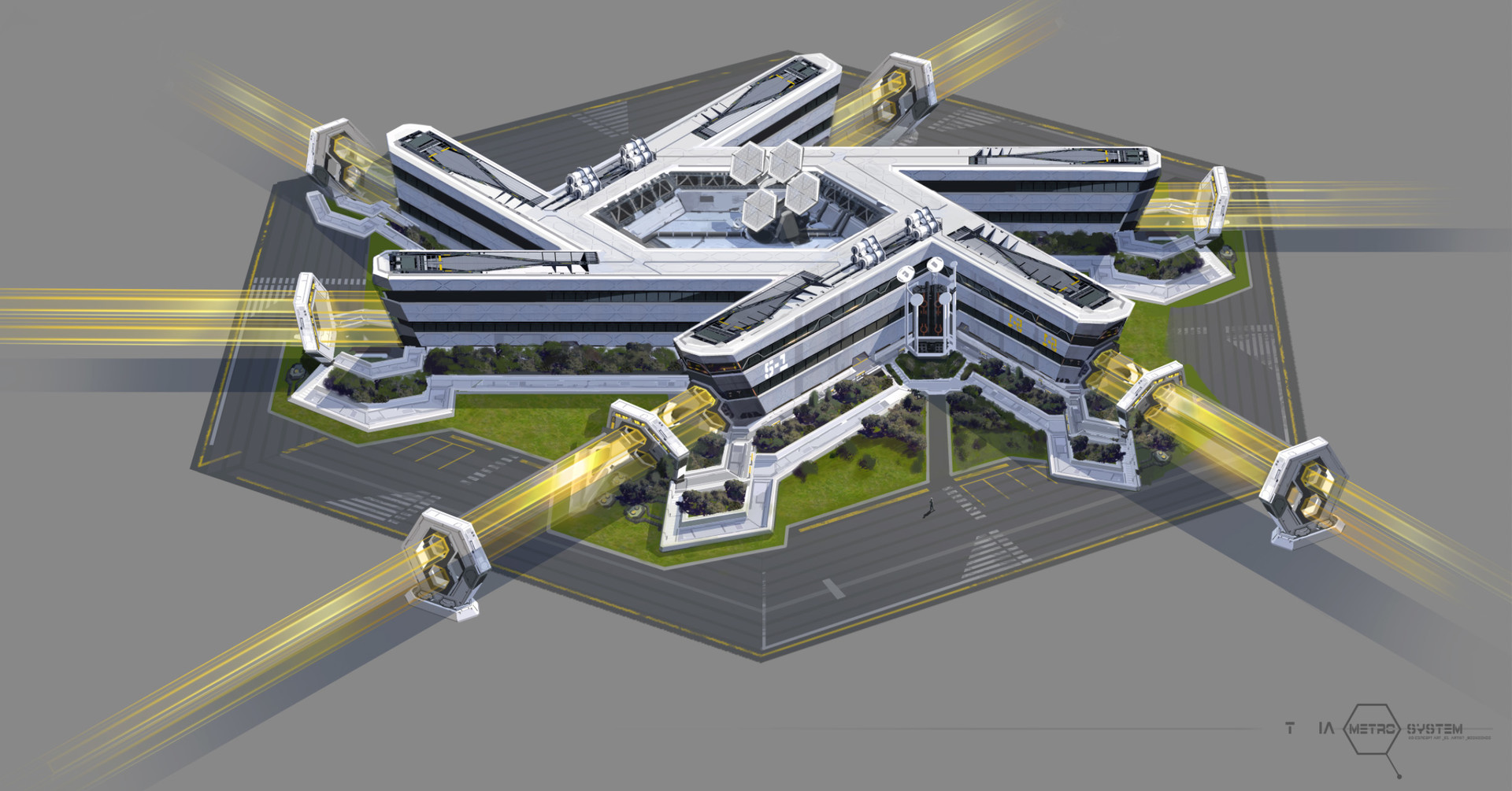This image is a highly detailed, computer-animated 3D color rendering of a futuristic transportation terminal. The terminal, primarily white and spanning four stories, features a unique, multi-sectioned design with segments angling off in different directions from a central structure. The background is a light gray hue, adding contrast to the building. Surrounding the structure are numerous windows, walkways, and a sidewalk, enhancing its modern appearance.

The building's form resembles a series of overlapping, metallic popsicle-stick shapes. At the base of the building, a gray hexagon encloses a grassy area. The roof showcases hexagonal panels, possibly solar panels, projecting upwards from a central cut-out area, reminiscent of a deep swimming pool without water. Golden light beams emanate from the central building, starting from hexagonal shapes and passing through the terminal, creating tunnel-like passages for transportation. There are six of these beams in total, three on each side.

This terminal is further surrounded by small trees and a well-maintained grassy expanse, blending nature with advanced technology. A dark gray graphic with a hexagon containing text, "Metro," marks the bottom right corner, indicating a transportation system integrated into this avant-garde structure.